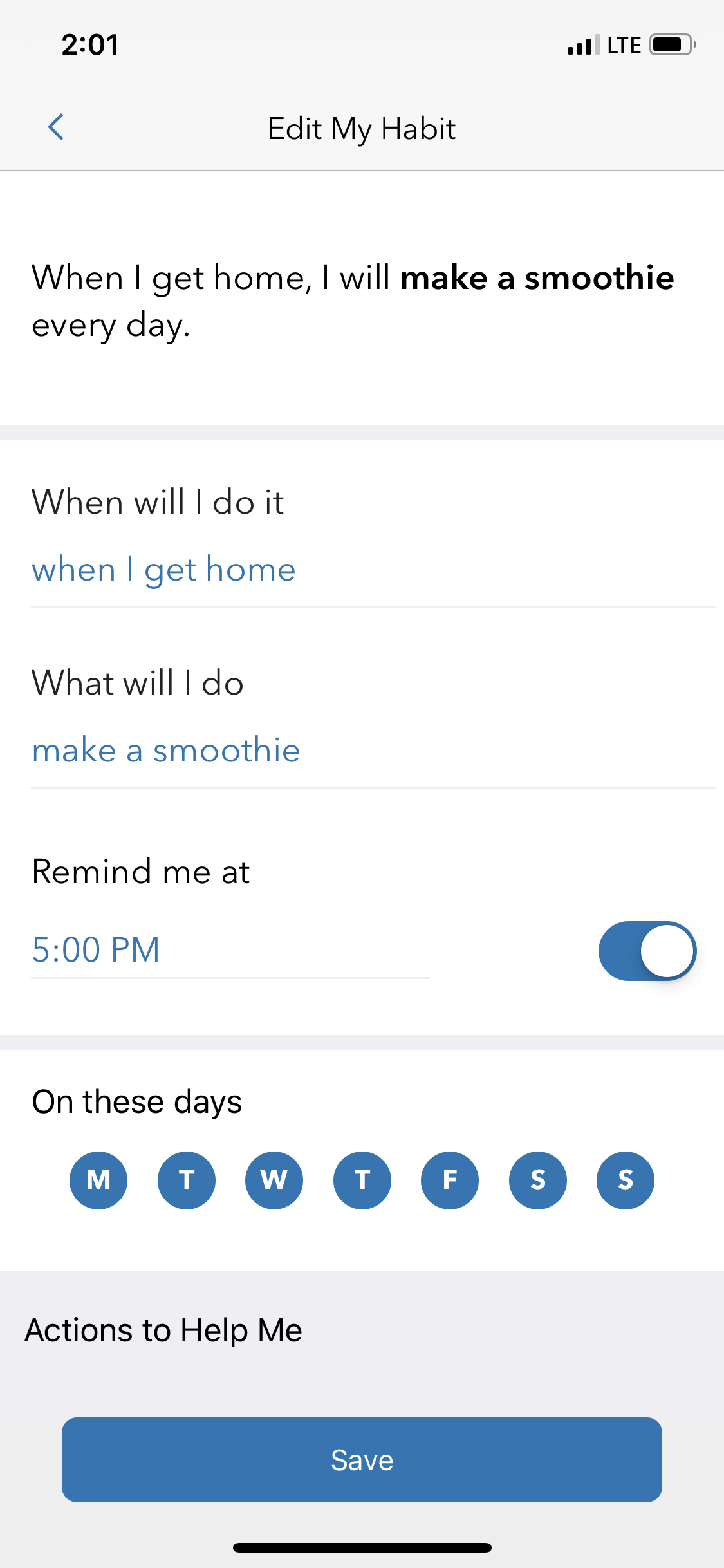A screenshot from an Android phone interface displays a structured habit tracking application. At the top, a light gray banner includes "201" on the left, signal strength with three out of four bars, "LTE," and a nearly full battery icon on the right. Below, an arrow pointing left precedes the centered text "Edit My Habit."

The primary section details a specific habit: "When I get home I will make a smoothie every day," with "make a smoothie" bolded. Beneath, a gray line marks a new section: "When will I do it?" with "When I get home" highlighted in blue. Another thin divider leads to "What will I do?" where "make a smoothie" is also highlighted in blue.

The following section, separated by another line, is titled "Remind me at" and specifies "5 p.m." with the toggle switch appearing to be on. The days of the week—represented by their first initials, M, T, W, T, F, S, S—are all highlighted, indicating daily reminders.

At the bottom, the section "Actions to help me" concludes with a "Save" button, ready to finalize the habit details.